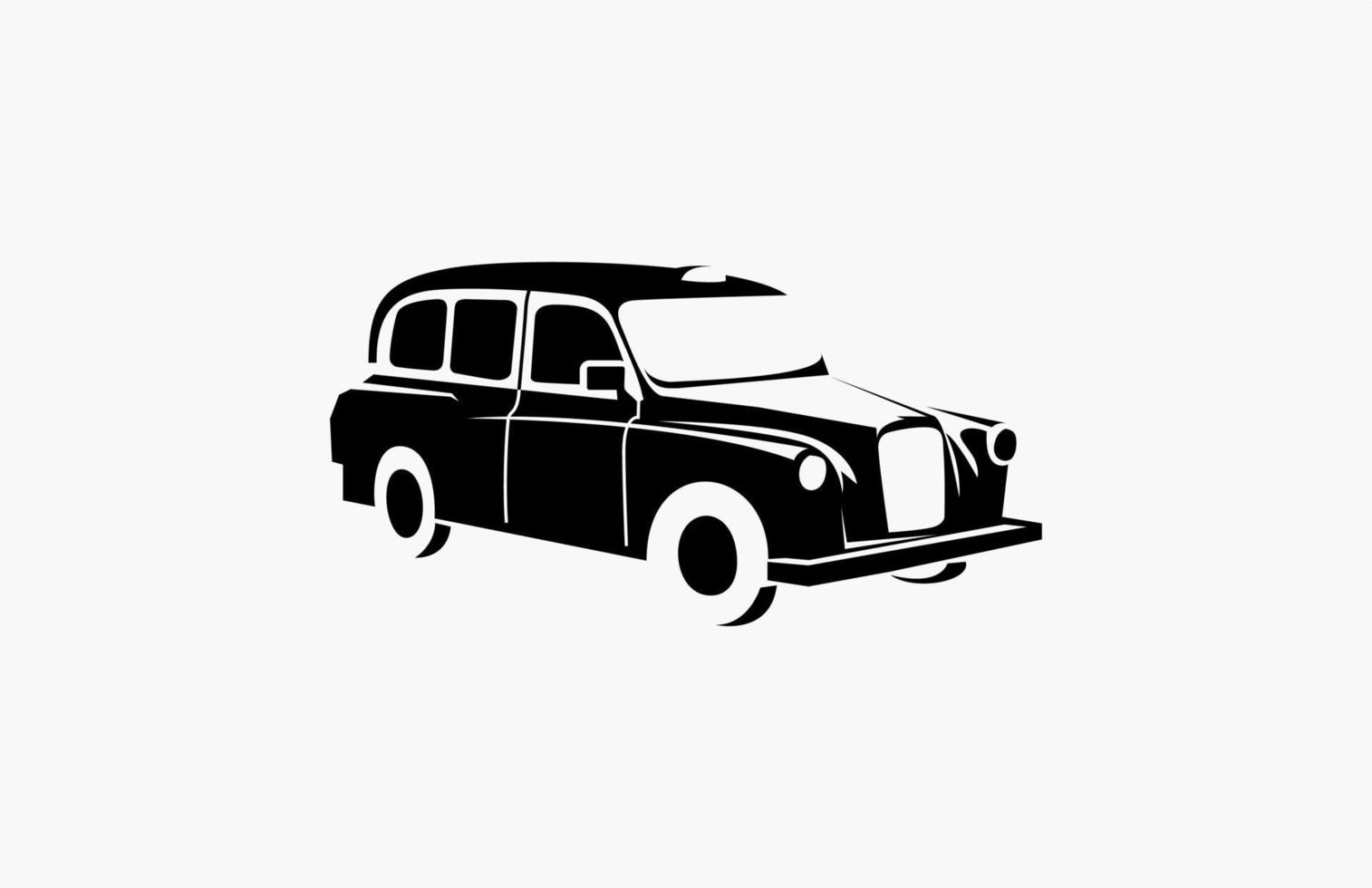The image is a horizontal rectangular drawing of a vintage car, depicted in a black-and-white color scheme. The car, evocative of 1940s or 50s design, possibly resembling an old Ford Hudson or a traditional taxi, is solid black with striking white accents. The background is a light gray, offering a clear contrast to the car. Viewed from a right front angle, key features include white-bordered black windows, a white windshield, and a white hood top. The vehicle’s distinctive grill is also white, flanked by asymmetrical headlights—one black and one white. The tires feature black centers and white walls. Notably, there's a small light on the roof indicating it might be a taxi. The simple, cartoon-like style of the drawing enhances its nostalgic, vintage appeal.